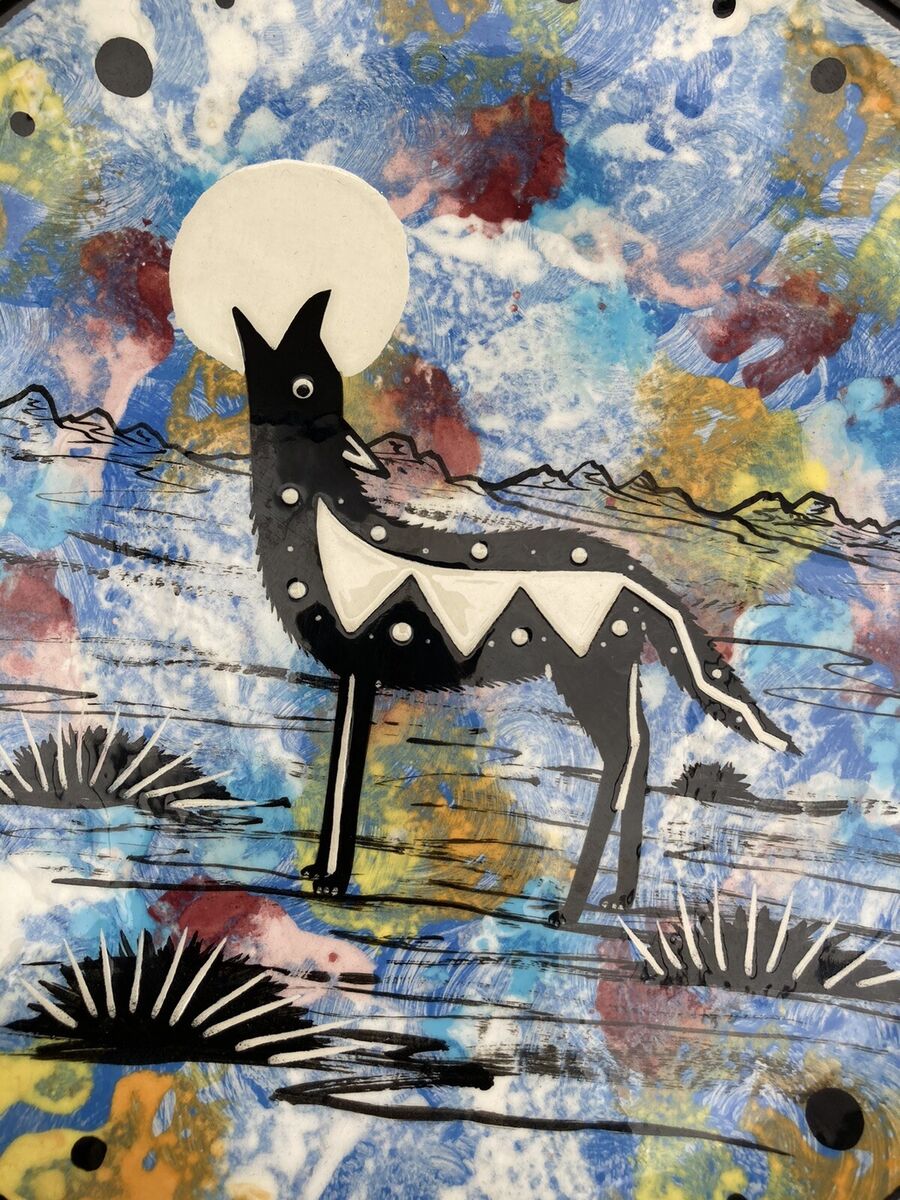The artwork depicts an abstract scene centered around a black and white wolf howling at a full moon. The wolf, positioned in the middle of the painting, has its head tilted upward with its mouth open, showcasing various white markings, including dots, stripes on its legs and tail, and triangular shapes. Surrounding the wolf are three bush-like, spiky objects in black and white, with two on the left. The background is a vibrant mix of blues, reds, yellows, and whites, featuring splotches and black dots, creating a dynamic and colorful setting. In the distance, black shapes resembling mountain tops add depth to the composition, emphasizing the wolf as the focal point of this vivid and imaginative piece of art.